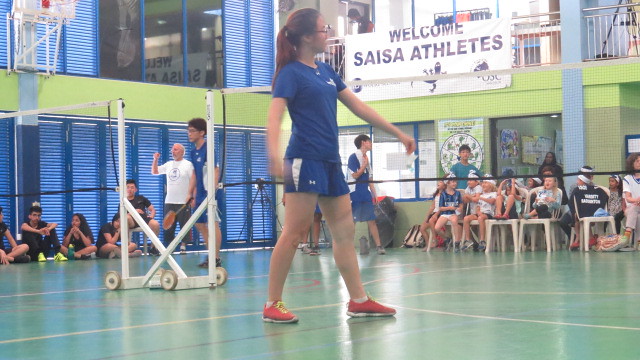In this vibrant indoor scene set within a school gymnasium, the photograph captures the energy of a sporting event. The gym floor is a striking green with beige markings, framed by blue dividers and green walls. Center stage stands a young woman, approximately 13 to 15 years old, with brown hair tied back in a ponytail, glasses, a blue t-shirt with white writing, and blue shorts with a white stripe down the side. She is outfitted with white socks and red sneakers. Her hands are extended, and she glances toward the top right corner of the frame, suggesting she is in the midst of a sports activity, likely volleyball given the visible net in the background.

The backdrop is bustling with activity; to the left, a group of younger children, about 6-8 years old, sit on white chairs, dressed mostly in shorts and appearing curious and engaged. More students, including a boy her age in similar attire and a man in a white t-shirt, sit directly behind her on the floor. Above them, a banner reads "Welcome SAISA Athletes" in blue letters, suggesting a special event or tournament. Further adding to the scene's depth, a balcony or mezzanine with a railing and several windows are visible, along with shaded doors, adding layers to the dynamic setting. The white item with wheels, a distinctive feature on the right side of the image, adds to the impression of an organized sporting event, reinforcing the photo's lively and bustling atmosphere.